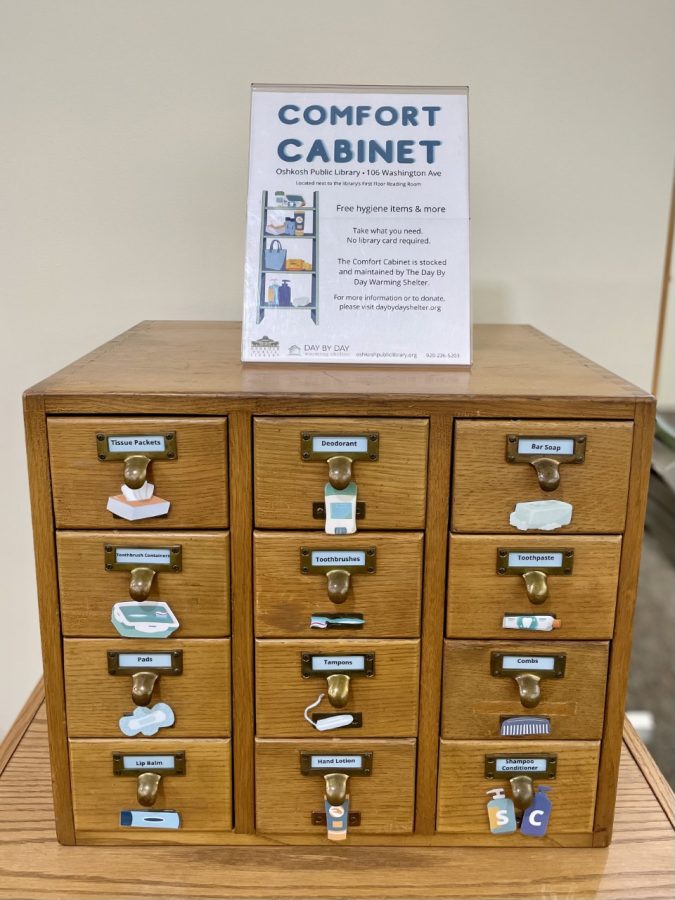This image showcases a light brown wooden cabinet, featuring a grid of 12 small drawers arranged in four tiers vertically and three tiers horizontally. Each drawer is equipped with a brass-colored knob and a label indicating its contents, although the specific names are unclear. Atop the cabinet, a sign with the words "Comfort Cabinet" is displayed in blue on a white background, accompanied by a standard-sized placard detailing information about the cabinet. The entire setup is situated on another light wood table, set against a white wall. This multifunctional cabinet appears ideal for organizing small items, making it a practical addition to any home or office.